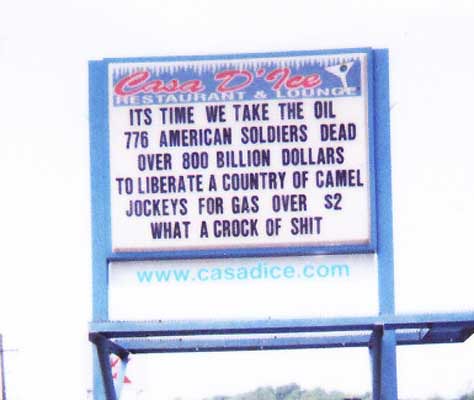The image captures a blue signage, held up by matching blue metal poles, in a first-person POV style with the camera tilted upwards. The bright, almost washed-out sky dominates the background, likely indicating the direction of the Sun. At the bottom of the image, a tree line is barely visible along with the tip of a power pole at the bottom left.

The sign features several key elements:
1. **Top Banner:** In a red script font, it reads "Casa de Ice," accompanied by a small graphic of a martini glass.
2. **Subheading:** "Restaurant and Lounge" appears in white text beneath the establishment name.
3. **Main Message:** Displayed on a white background with blue text, it reads, "It's time we take the oil. 776 American soldiers dead. Over $800 billion to liberate a country of camel jockeys for gas over $2. What a crock of shit."
4. **Footer:** The web address "www.casadeice.com" is shown at the bottom.

The image appears to be of mediocre quality, possibly scanned or re-photographed multiple times, contributing to its blown-out and bright appearance.